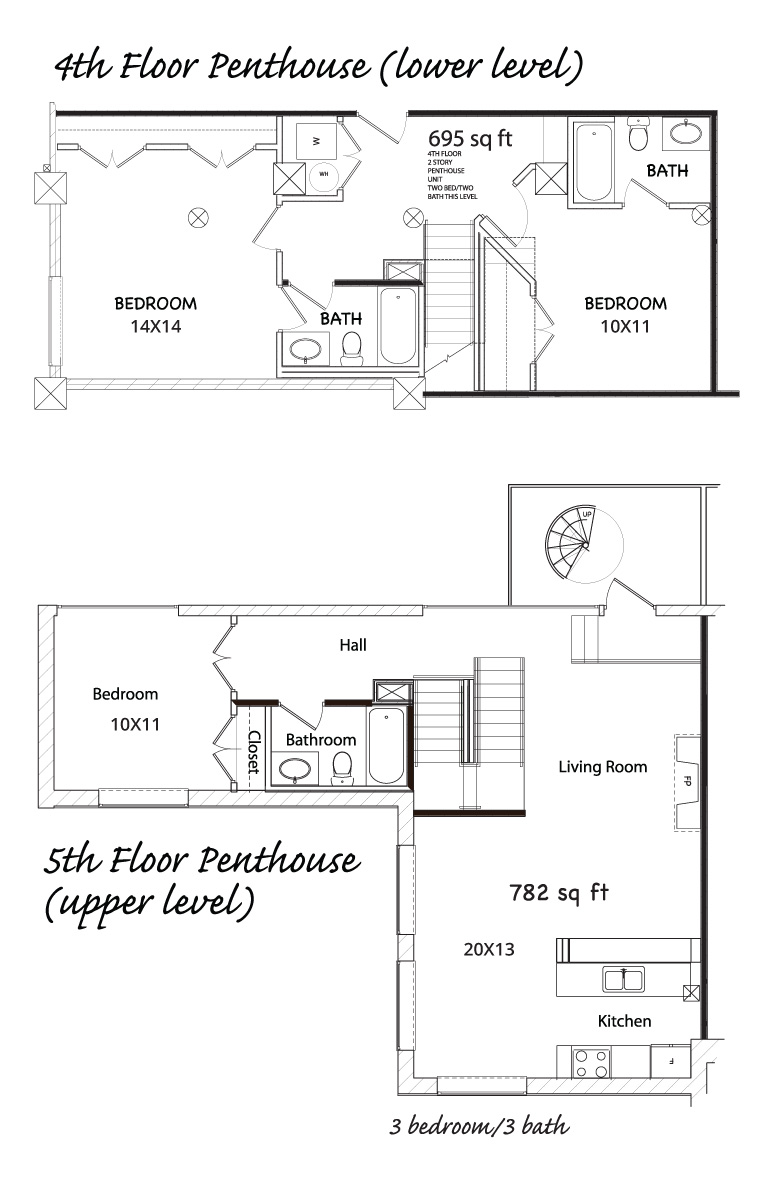**Detailed Penthouse Floor Plan Description:**

The image depicts a detailed floor plan of a two-story penthouse, encompassing the fourth and fifth floors of the building.

**Fourth Floor Penthouse (Lower Level):**
- The top half of the illustration is labeled "Fourth Floor Penthouse" with a note in parentheses indicating it is the lower level.
- On the left side, there's a bedroom measuring 14 by 14 feet. This bedroom has a doorway leading to an adjacent bathroom at the lower section of the plan, which contains a bathtub, toilet, and sink.
- Moving upward, towards the front of the plan, there's a space designated for a washer and dryer, accessible through a door that presumably leads to the outside.
- In the central section, the space is labeled "695 square feet" with some illegible writing nearby.
- A staircase is illustrated, leading upwards to the next floor.
- Adjacent to the staircase, another bedroom is depicted, measuring 10 by 11 feet, with an attached bathroom located at the upper right corner of this bedroom.

**Fifth Floor Penthouse (Upper Level):**
- The bottom half of the plan is labeled "Fifth Floor Penthouse" indicating it as the upper level.
- The staircase ascends into a hallway that leads directly into another bedroom measuring 10 by 11 feet. 
- This upper level also includes a bathroom and closet adjacent to the bedroom.
- A spacious living room is shown, labeled "782 square feet" and measuring 20 by 13 feet. This room appears to feature a fireplace situated along the side wall.
- The kitchen is positioned in the upper right corner of the plan.
- Overall, the fifth-floor layout summarizes the penthouse as containing three bedrooms and three bathrooms.

This detailed floor plan provides a comprehensive overview of the two-story penthouse, highlighting its layout, room sizes, and key features.